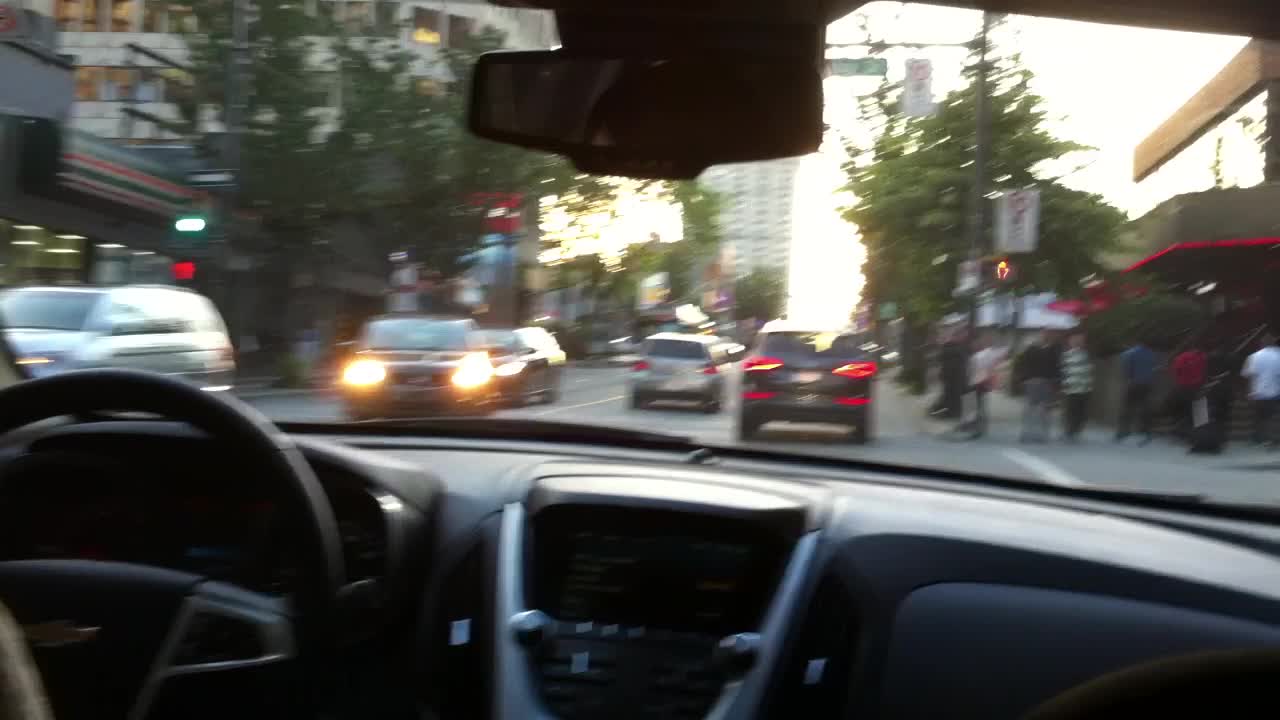This is a photograph of a slightly blurry, urban traffic scene taken from inside a vehicle. The image captures a black and silver dashboard with a centered media area comprising knobs for volume and air conditioning, flanked by air vents. The black steering wheel is visible in the bottom left corner without any hands on it. The rearview mirror is situated at the top center of the image. Outside the front windshield, it's either early morning or approaching evening as suggested by the dim lighting. The car is in the right lane, following two other vehicles traveling in the same direction. Opposite traffic shows several cars with headlights on. To the right, a group of people is gathered near a crosswalk with a red stop hand signal, likely entering a nearby building. On the left side, several vehicles are heading in the opposite direction, along with buildings, including a recognizable 7-Eleven with its distinct striped banner. In the background, a tall corporate office building is illuminated by the setting or rising sun, providing a striking contrast against the urban setting.